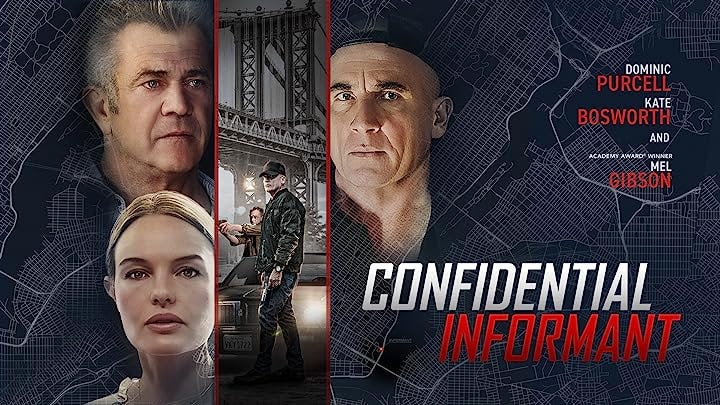The image is a detailed movie poster for "Confidential Informant," prominently displaying a black-and-white illustration of New York City, featuring landmarks like Manhattan and Central Park. The poster is overlaid with the large faces of three main actors: Mel Gibson in the top left, Kate Bosworth in the bottom left, and Dominic Purcell on the right. In the center, below the actors' faces, there's a cutout strip showing Kate Bosworth and Dominic Purcell under the Manhattan Bridge, each brandishing a gun—Kate behind a car, and Dominic in front, looking out in the distance. The title "Confidential Informant" stands in bold at the bottom right, with "Confidential" in white and "Informant" in red, both italicized and in all caps. Above the title, the actors’ names are displayed, also in white and red, with Mel Gibson uniquely highlighted as "Academy Award winner Mel Gibson." The overall layout enriches the visual narrative, emphasizing the film's suspenseful tone.